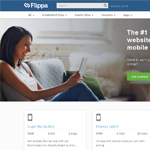This is a description of the blurry screen capture:

In the image, there is an interface with a blue header featuring a logo that is likely "Flippa" (spelled F-L-I-P-P-A). Next to the logo, there is a search field. The menu appears to be grayed out due to the blurriness, displaying five options. Below the header, there is a hero image of a woman sitting comfortably on a couch. She has medium-length hair, and is wearing a sleeveless white top paired with jeans. She is either holding a phone or an iPad, with her legs bent and hands resting on her knees. Cushions are placed on the couch, and in the background, there is a window on a white wall.

To the right side of this hero image, some text is partially visible. It begins with "the number one website, mobile..." and appears to be accompanied by a green button, presumably labeled "Get Started." Below the main white text, there is additional subtext. Underneath the image, there are two phone icons, which seem to suggest options for ordering a phone, accompanied by descriptive text in blue. Further down, the layout displays more detailed text separated by spaces, along with some general information. The overall background of the interface is white.